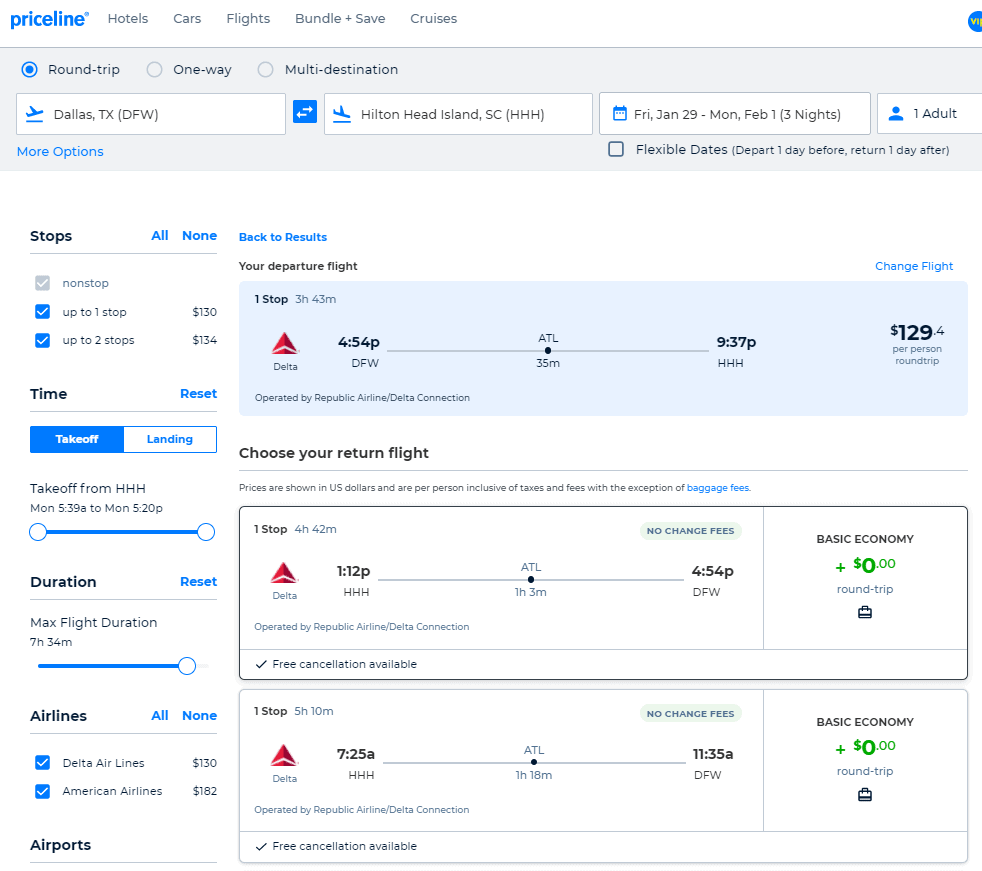The image captures a computer screen displaying travel booking details on Priceline for a trip from Dallas, Texas to Hilton Head Island, South Carolina. The itinerary shows a departure from Dallas with arrival in Hilton Head on Friday, January 29th, and a return on Monday, February 1st. The booking is for one adult and specifies that the departure flight includes one stop. The screen details the flight times, indicating both the departure and landing schedules. It outlines the pricing options: a flight with up to one stop for $130 and up to two stops for $134. The viewer can choose a return flight and is presented with a basic economy option, which includes no change fees. The travel duration for options with one stop is specified as 4 hours and 42 minutes. Additionally, the screen highlights a round-trip basic economy fare, listing the total cost as $0.00 in certain areas. This setup page helps in planning the trip comprehensively.